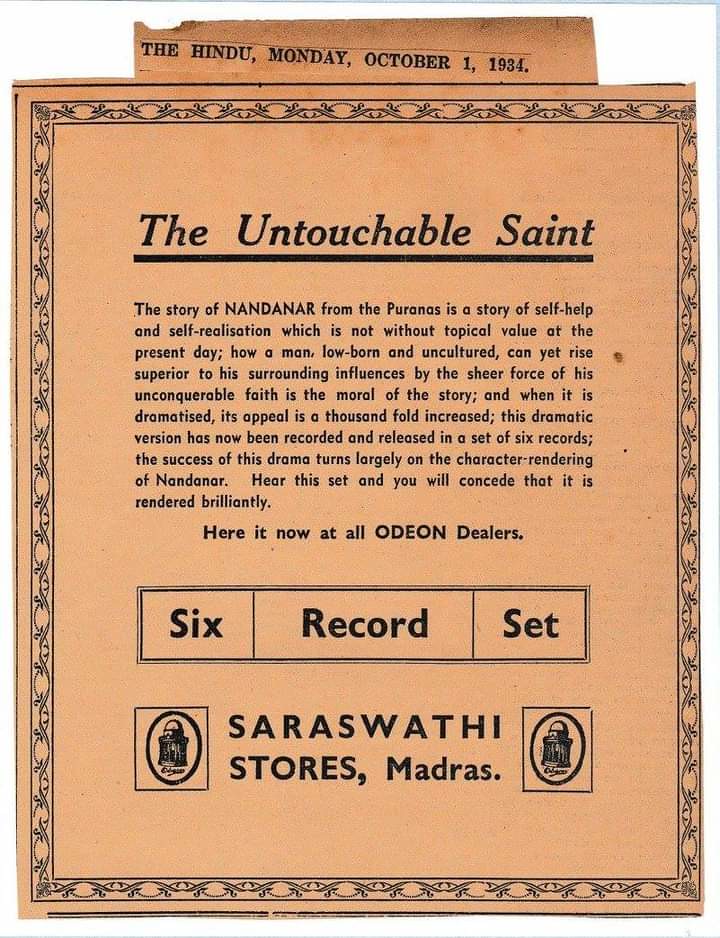The image is a rectangular flyer with a light brown, almost orange-ish background, adorned with an ornate vine-like border. Attached at the top of the flyer is a separate strip that looks like it was added or taped on, reading "The Hindu, Monday, October 1, 1934" in black text. The central headline of the flyer is "The Untouchable Saint," which is prominently underlined. Below the headline, the flyer provides a background on Nandanar, describing his story from the Puranas as a tale of self-help and self-realization, highlighting how a low-born, uncultured man rises above his surroundings through the strength of his faith. This narrative has been dramatized and is available as a set of six records. The flyer encourages readers to hear this brilliant rendition at all Odeon dealers. A rectangular box at the bottom of the flyer emphasizes "Six Record Set," and below this, it mentions "Saraswati Stores, Madras," alongside small logos on either side.